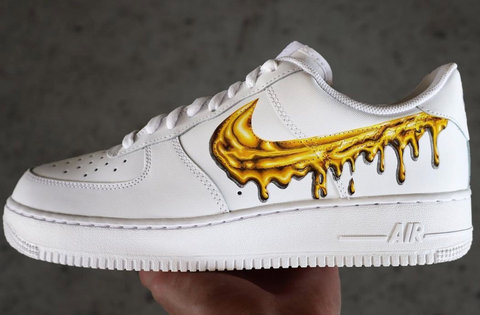The photograph features a close-up of a unique white Nike Air sneaker being held and presented from the side. The sneaker is predominantly white with white laces and a white sole, which has the word "Air" embossed in white at the heel. The most striking feature of the shoe is the gold Nike Swoosh on its outer side; the swoosh has a dripping effect, making it appear as though it is made of molten gold or wet paint. The sneaker is held by the palm of a person's hand, which is partly visible at the bottom of the frame. The backdrop is a dark, speckled gray, adding contrast and drawing attention to the sneaker's clean lines and unique design details.